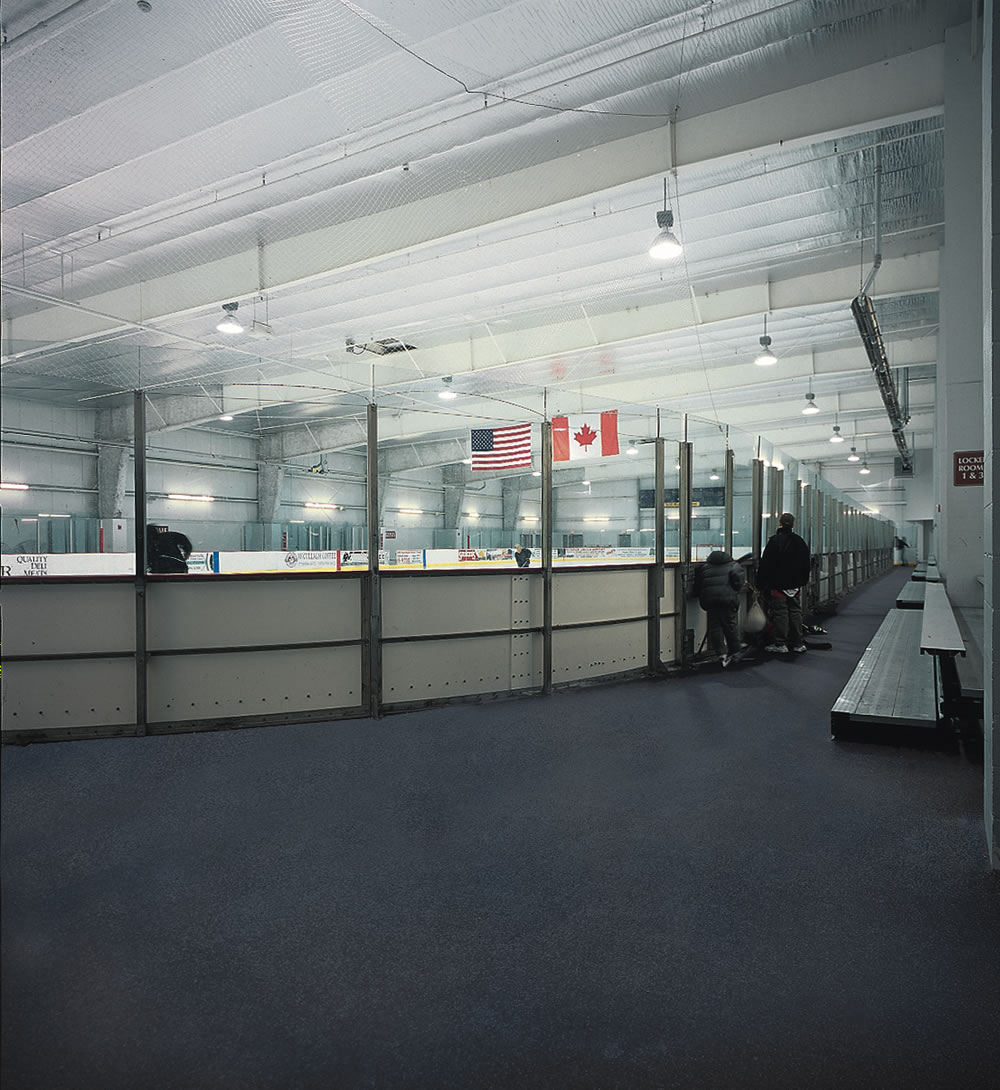This photograph captures the viewing area outside of a hockey rink situated within a large indoor stadium. The expansive ceiling, adorned with shades of white, is supported by giant steel girders and dotted with fluorescent lamps and air ducts. Dominating the scene, an American flag hangs to the left while a Canadian flag hangs to the right from the rafters. The hockey rink itself features a sturdy boundary: the lower half is lined with white steel panels, while the upper half is enclosed by clear glass or hard plastic panes supported by steel bars. To the right, a series of steel bleachers are lined up against the wall, providing seating for spectators. The dark gray carpeted flooring supports a couple of onlookers standing outside of the rink, watching the hockey players glide across the ice as they engage in the game.